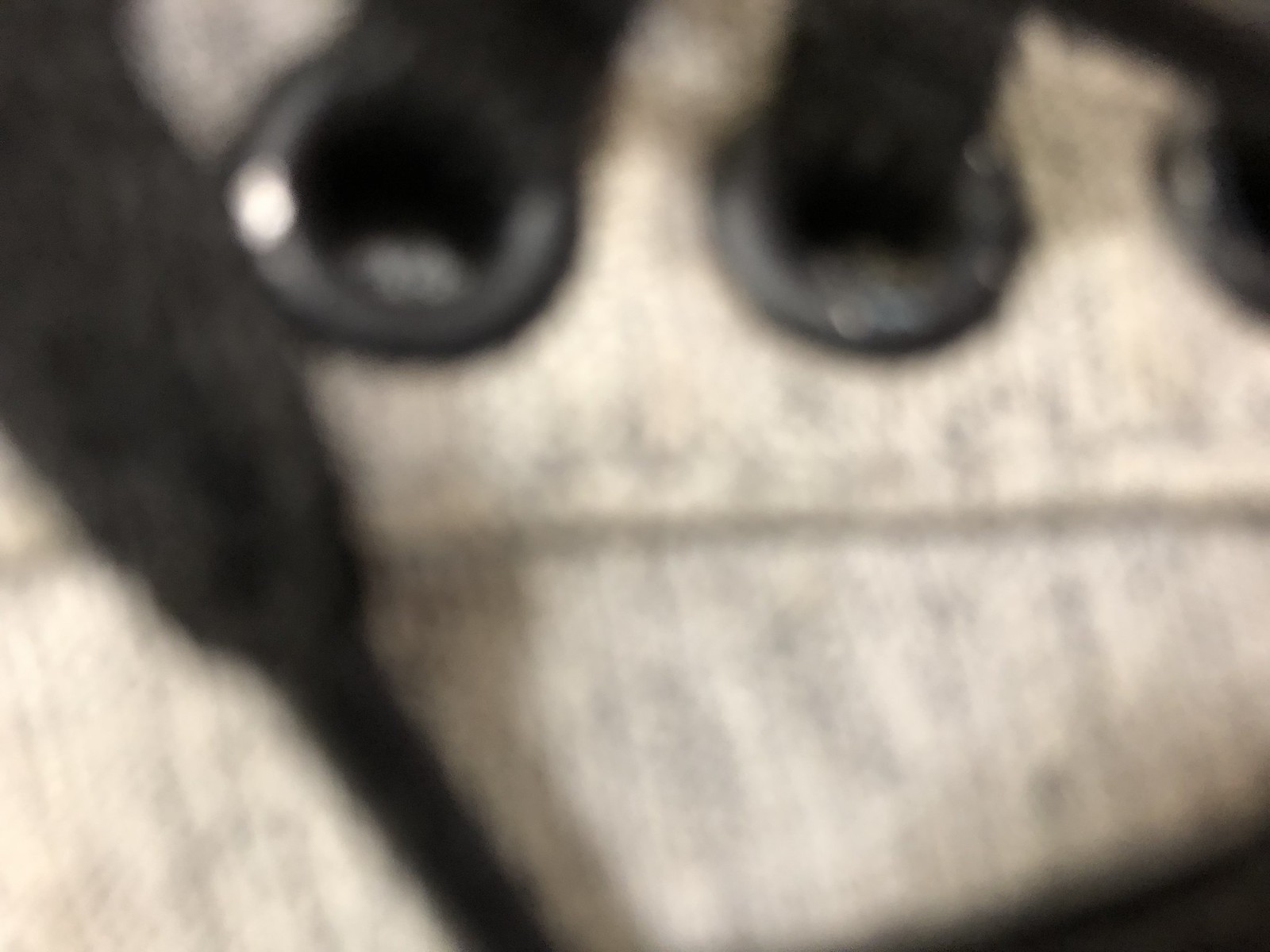This image depicts a highly blurred and abstract scene, featuring a predominantly black background. Dominating the center is a large, indistinct white and gray rectangular area. Within this area, there are two prominent black circular shapes situated near the top. Emerging from these dark circles are what appear to be black protrusions or poles. The overall composition, with its close-up nature and lack of sharpness, resembles the top section of a grommet curtain through which a curtain rod would be inserted. However, the extreme blurriness makes definitive identification of the objects challenging.